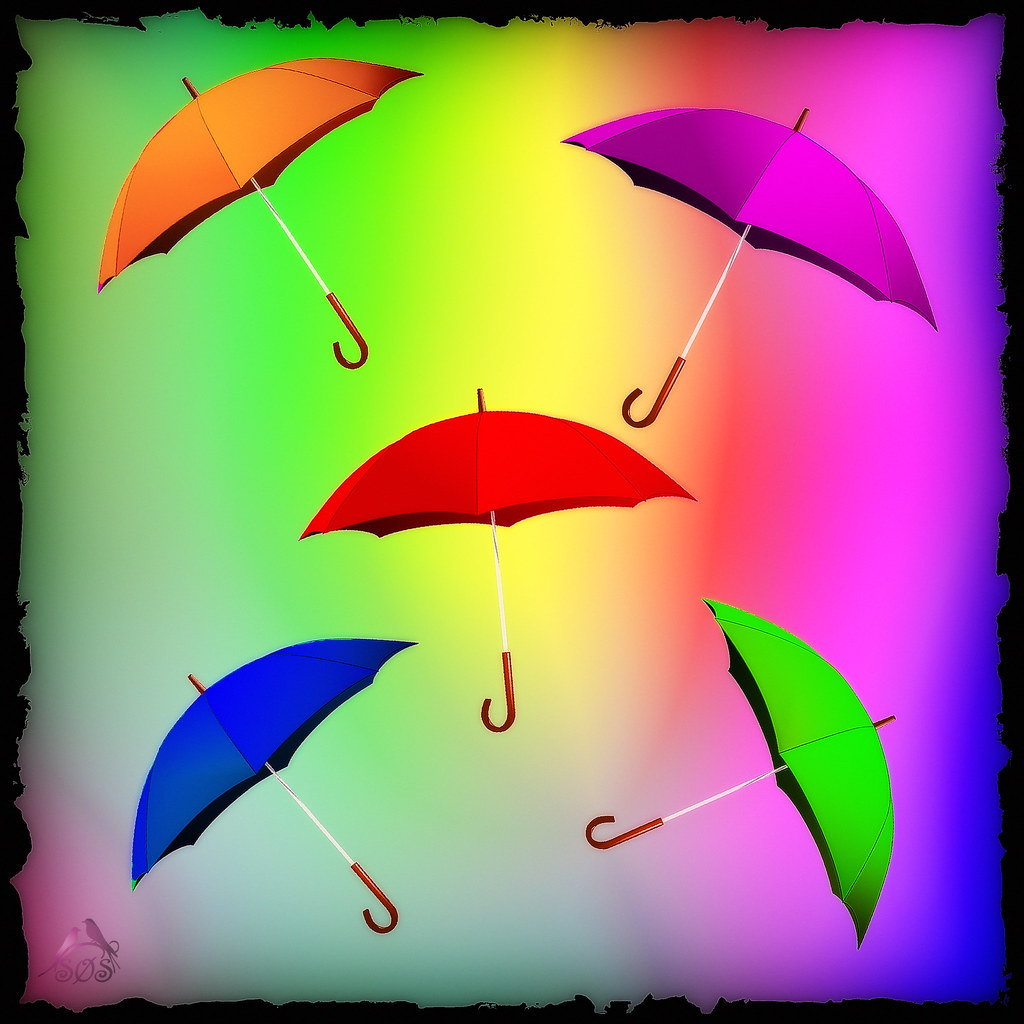This detailed illustration features five umbrellas and a vibrant rainbow gradient background. Each umbrella, identical in design but varying in color, has a J-shaped wooden handle. Centrally positioned is a red umbrella. To its left at the top, an orange umbrella tilts leftward, while directly opposite on the right, a purple umbrella tilts rightward. On the bottom left, there's a blue umbrella also tilting left, and on the right, a green umbrella tilts right. The background transitions seamlessly through a spectrum of colors: green, dark green, yellow, red, purple, and blue. At the bottom left, the letters "S.O.S" appear in an enchanted, fantastical font, accompanied by silhouettes of two birds facing each other. The entire illustration is framed by a simple black border, enhancing the overall textured and colorful appearance of this graphic design piece.